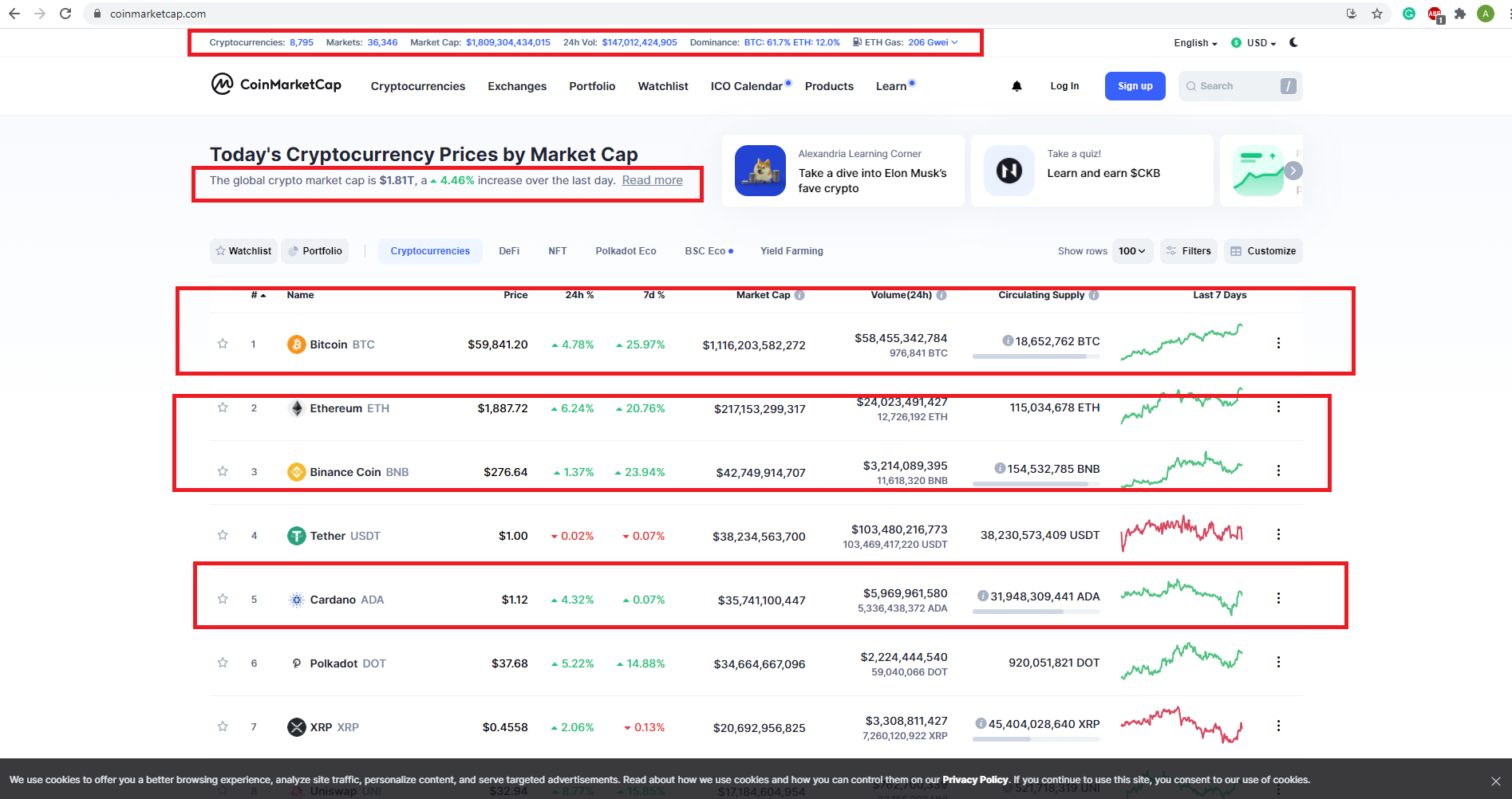This image is a screenshot taken from the CoinMarketCap website, capturing a heavily loaded web page filled with comprehensive cryptocurrency information. The screenshot, with a small file size, somewhat obscures finer details but still offers a clear view of the layout and content. The web address bar at the top indicates the URL: coinmarketcap.com. Several sections of the page are highlighted with red rectangular boxes, focusing attention on specific areas.

At the top of the page, there is a prominently displayed list of cryptocurrencies, accompanied by various statistics including market capitalization. The website features a navigational menu that offers quick access to pages for cryptocurrencies, exchanges, portfolios, watchlists, ICO calendars, products, and educational resources under the 'learn' section. Additionally, options for logging in and signing up are conveniently located in the right-hand side menu.

The main content of the page presents today's cryptocurrency prices categorized by market cap, displayed in a neat, table-style format. Each row in the table lists different coins along with multiple columns of data, including a seven-day trend line chart, providing a visual representation of each cryptocurrency's performance over the past week.